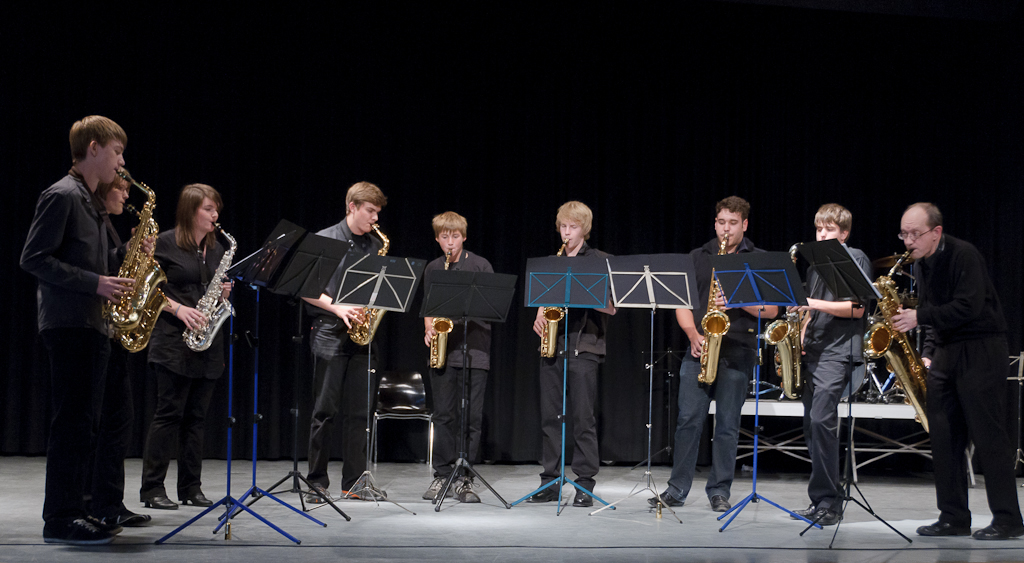The image depicts a school band, composed predominantly of male students, situated on a stage with a gray floor and a black backdrop. The musicians are part of a trombone section, each dressed uniformly in black outfits consisting of long-sleeve shirts, pants, and shoes. They are standing semi-circle, each behind a music stand—most of which are black, though a few are blue and one is white. 

From left to right, specific individuals stand out: a boy in a gray shirt and black pants plays the trombone, partially obscuring a girl's face who matches the black outfit uniform. Adjacent to her is another girl with long brown hair, also playing a trombone. Beside her, slightly to the back, is a boy facing right with short brown hair. Next in line is a shorter boy with blonde hair facing the camera, followed by a taller boy with really blonde hair, also positioned towards the camera. Another boy to the right, with short brown hair, is playing a trombone, facing forward. Further to the right, stands yet another boy with short brown hair similar to his counterparts, playing his trombone while facing the camera. On the far right is an older, balding man with glasses, likely the teacher. He stands slightly leaned over, holding a larger trombone and dressed similarly in a long-sleeve black shirt and black pants. In the background to the right, a distant stage is dimly visible.